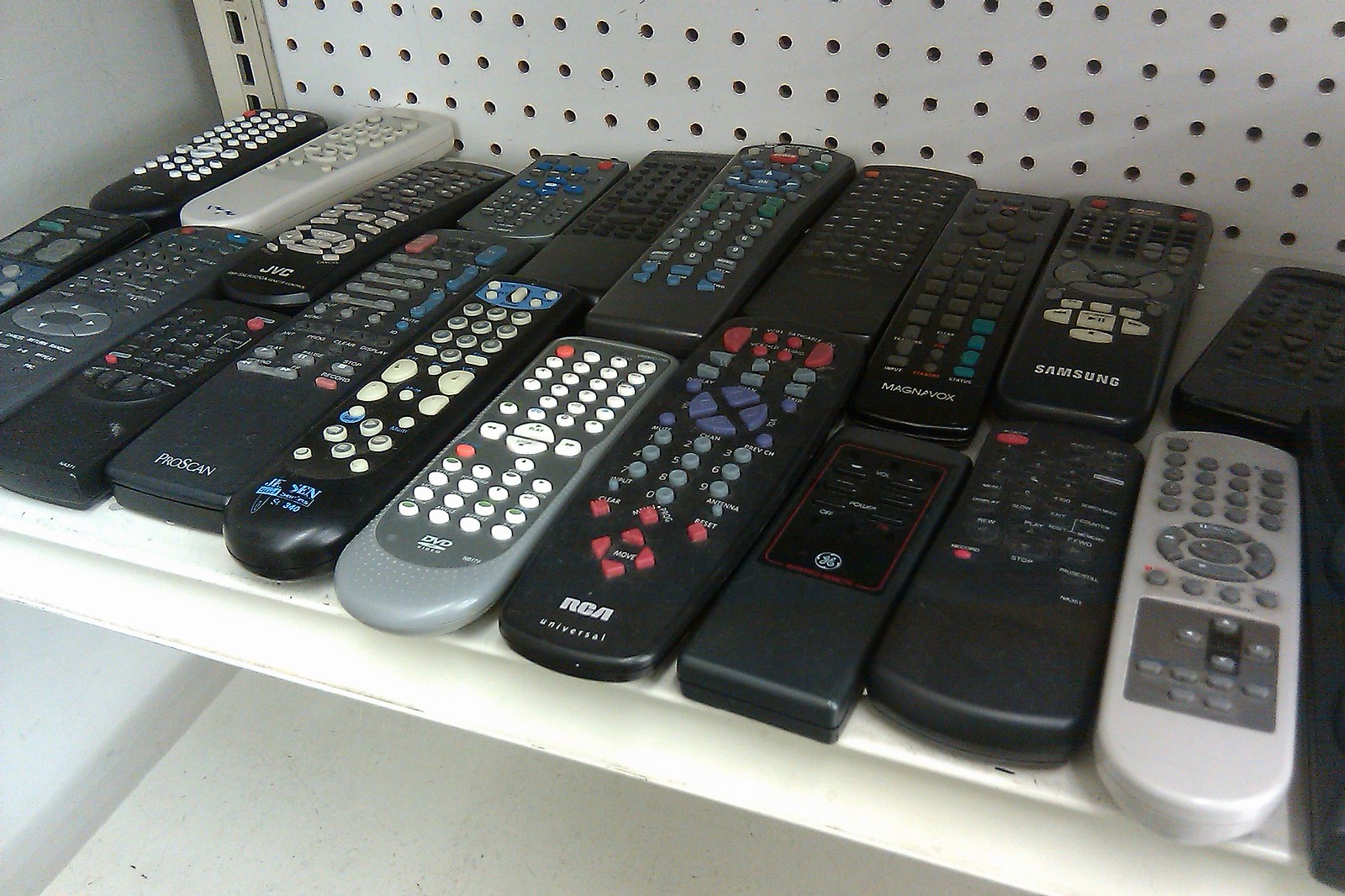This close-up horizontal photograph captures a store shelf display of various television remote controls. The scene is set against an ivory-colored metal shelf with a curved inward edge, mounted on a pegboard type backing. Another shelf is visible beneath it, but it is empty. The remote controls are meticulously arranged in one or two rows, some stacked one above the other. The remotes vary in color, ranging from black to various shades of gray, and even tan. The buttons on these remotes feature a mix of white, red, gray, and blue. Brand logos such as RCA, Samsung, Magnavox, and ProScan are noticeable at the bottom of several remotes, indicating they are for older CRT televisions. The detailed buttons and brand variety signify a range of functions and compatibility with various vintage TV sets.